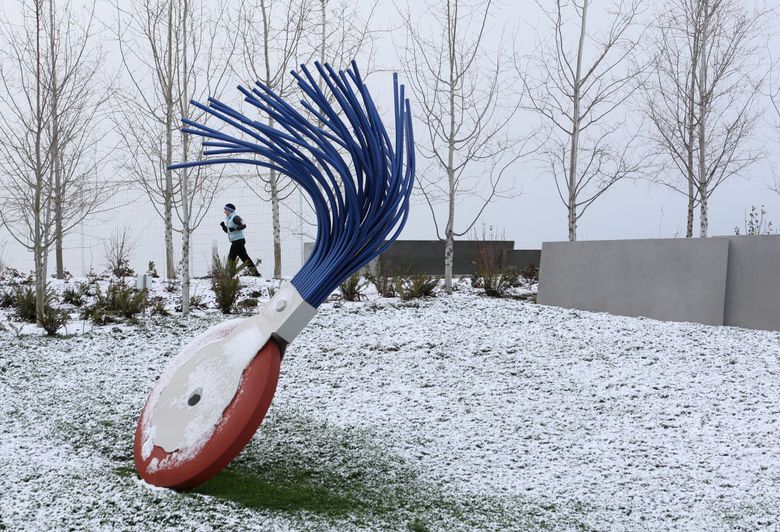In this outdoor color photograph taken during a gray winter day, a light dusting of snow covers the ground, faintly blanketing the grass and hinting at the season’s early snowfalls. The background features a row of thin, bare trees, with a jogger dressed in black pants, a black long-sleeved shirt, a pale blue vest, winter mittens, and a hat, jogging towards the left on what appears to be a walking path. The scene is framed on the right by a concrete wall, possibly part of a municipal or college building, and some bushes underneath the trees. The focal point of the image is a striking outdoor sculpture set in the center of the photo. The sculpture resembles an old-fashioned pencil eraser designed as a large, dark red, wheel-shaped base coated lightly in snow. Emanating from this wheel is a rectangular metal piece topped with blue, tentacle-like streamers pointing to the left, reminiscent of a brush meant to clear away eraser shavings. The sculpture, contrasting with the serene winter setting, adds an artistic touch to what is presumably a park-like area.